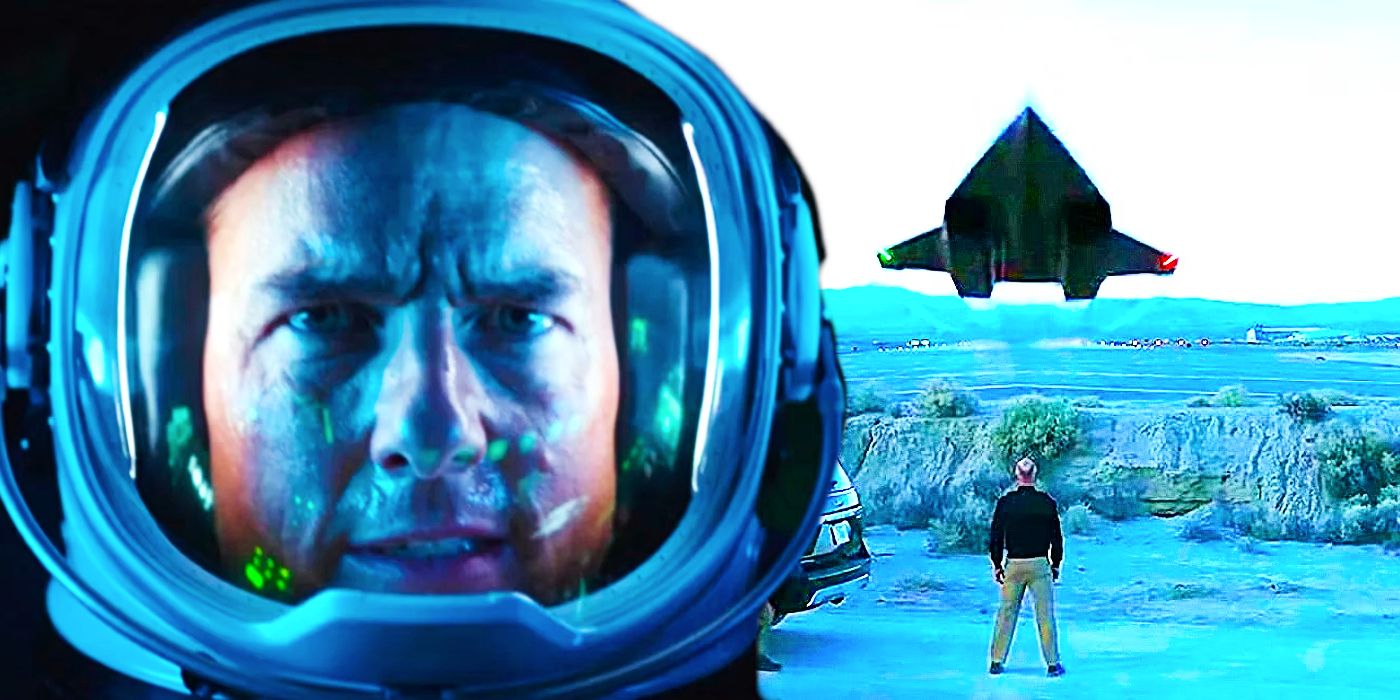This image, possibly AI-generated and resembling a scene from a space movie, features a striking juxtaposition of two distinct elements. On the left side, there is a close-up of a man resembling the actor Tom Cruise, encased in the helmet of a futuristic or astronaut suit. The helmet, glowing with a bluish hue, reflects various illuminated images, enhancing the sense of a high-tech environment. His face, sharply detailed with gritty determination, has a furrowed brow and parted lips, suggesting intense focus as he gazes forward. 

The right side of the image portrays a different man, standing on what appears to be barren land with a surreal, bluish cast. He is dressed in a long-sleeved black shirt and khaki pants, with a noticeable balding spot on his head. This man is looking upward, captivated by a large, unusual aircraft resembling a secret military plane or spaceship that hovers above. The background includes turquoise blue terrain with rocks, some sparse green vegetation, and possibly more aircraft in the distant fields. There is also a glimpse of a vehicle bumper near the man, adding to the scene's mystery and technological ambiance.